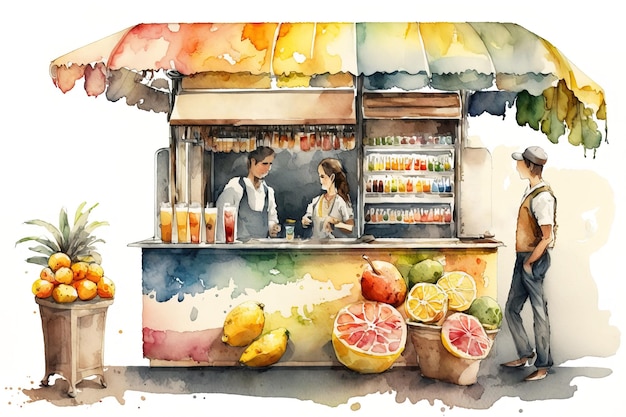This stylized watercolor painting depicts a quaint, tattered-canopy juice kiosk, with vibrant colors blending together in typical watercolor fashion. A young couple, dressed in white shirts and aprons, engage in conversation inside the kiosk, behind a small bar counter adorned with five tall glasses of colorful, frothy juice. The kiosk's exterior walls are decorated with paintings of various fruits including lemons, mangoes, watermelons, cantaloupes, limes, oranges, apples, and pears, creating a vibrant, eclectic display. On the left side, a stand showcases real fruits like large oranges and apples, while a square vase contains a pineapple tree stacked with mangoes. To the right, shelves hold an assortment of juices and equipment, some of which appear to be in a freezer. A patron, who appears to be awaiting service, stands nearby wearing a hat with a bill, a brown jacket, grey trousers, and brown shoes. His eyes are curiously absent, adding a unique touch to the painting. The overall scene is reminiscent of a small, colorful food cart, complete with a drapery overhang and a lively, bustling atmosphere.